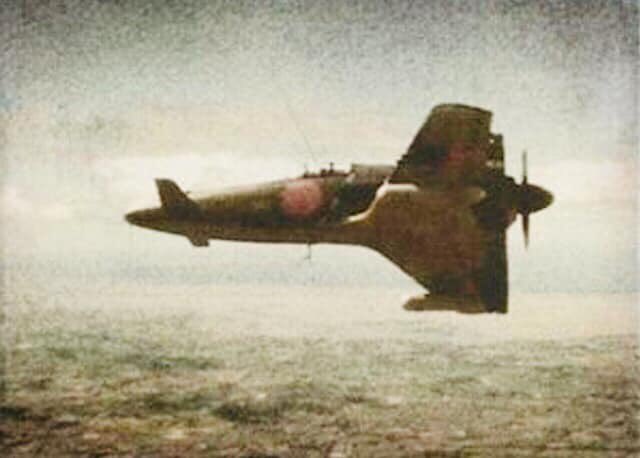This appears to be a very old, grainy photograph of a World War II-era Japanese airplane, characterized by its unique design and the distinctive faded red circle indicative of the Japanese flag on its fuselage. The image predominantly features brown, gray, and black tones, contributing to its worn and dated appearance. The plane, which has a propeller at the back, likely indicating it’s a rear-engine aircraft, is positioned centrally in the photo and appears to be flying over a landscape, though the ground detail is difficult to discern due to the graininess of the image. The wings of the plane extend in an unusual manner, almost appearing backward, perhaps distorted by the age and quality of the photograph. The background shows a mix of white and gray hues, suggesting either sky or an overexposed landscape. Despite the lack of clarity, the plane's historical design and aged condition vividly capture the essence of an era gone by.